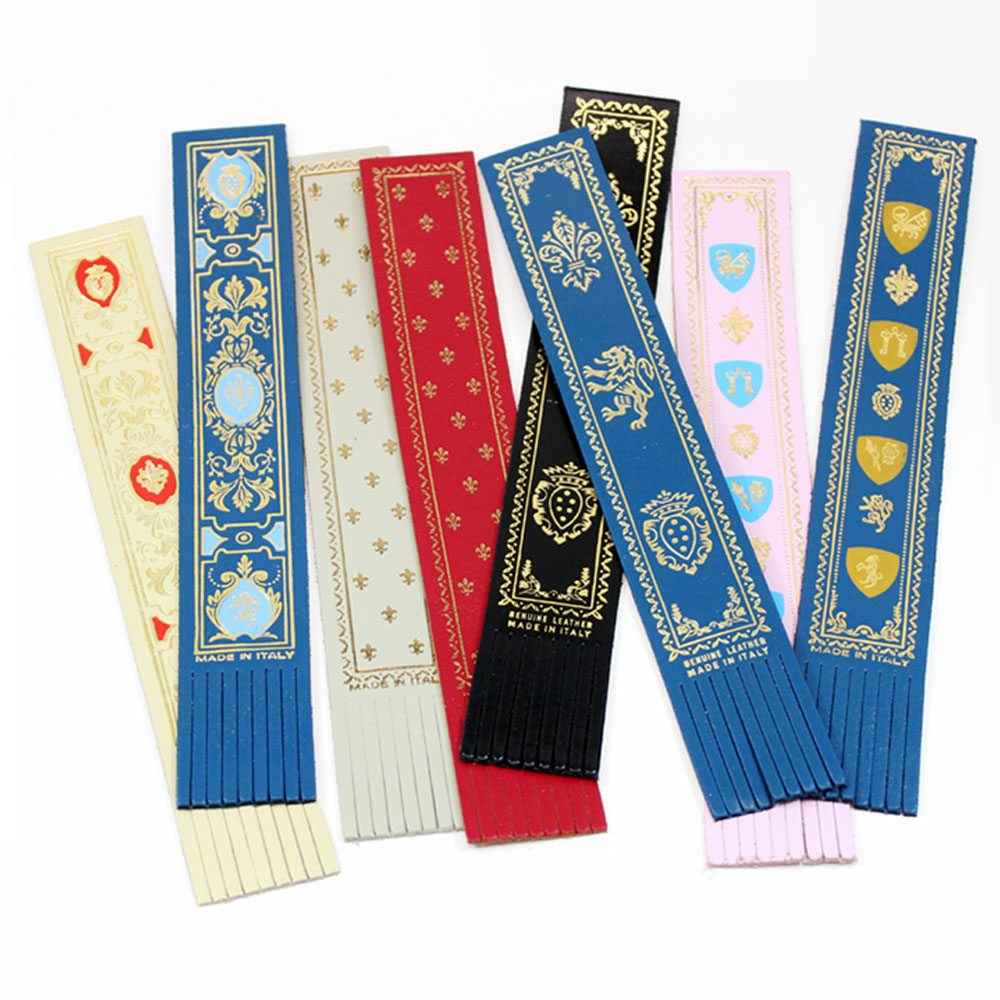This image showcases eight intricately designed leather bookmarks, each distinctly colored and adorned with unique patterns. Starting from the left, the first bookmark is milky in color with red designs on it, atop which lies a blue bookmark featuring golden flowery designs and the inscription "made in Italy." All the bookmarks have frayed edges that are uniformly cut, enhancing their crafted appeal. The next bookmark, also milky with a colorful design, contrasts with the subsequent red one adorned similarly. Following this is a black bookmark engraved with a gold pattern and marked with "made in Italy genuine leather." The collection includes three blue bookmarks, a pink one, and a light gold bookmark. Each bookmark displays an array of designs including delicate crest shapes, lions, shields, and fleur-de-lis emblems, indicating an artistic and possibly heraldic inspiration. The bookmarks are neatly arranged against a blank background, focusing all attention on their detailed craftsmanship and vibrant colors.